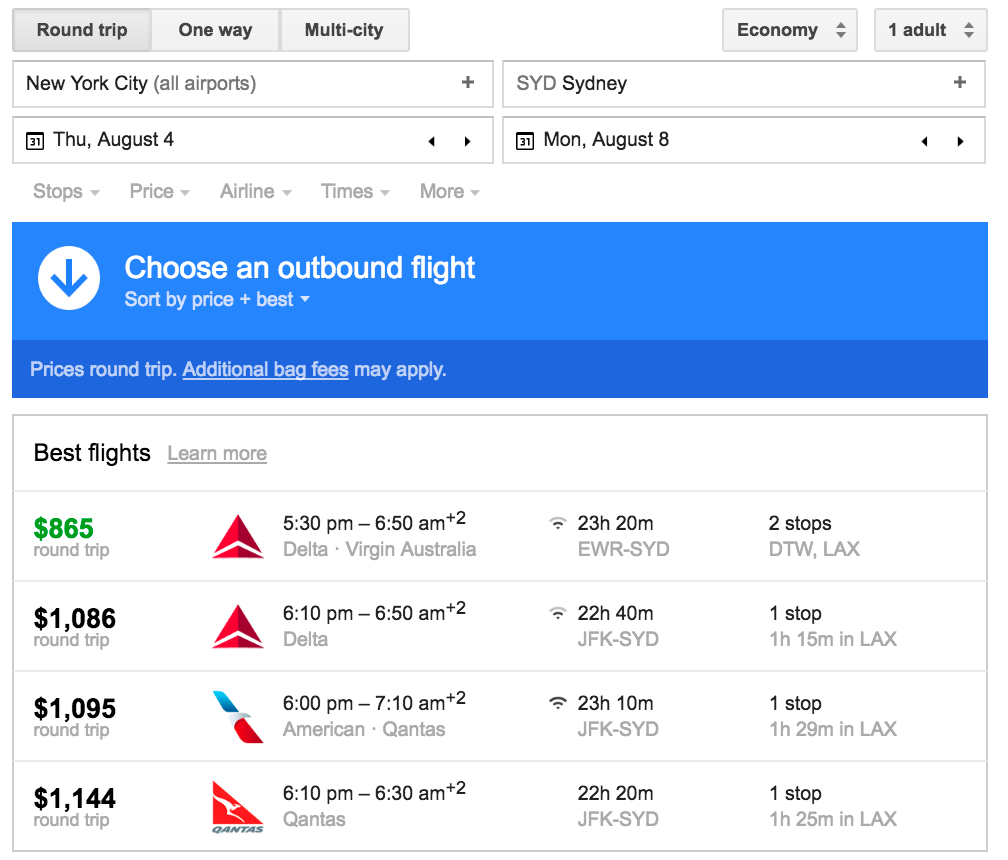In this image, we see a screenshot featuring a flight search interface set against a solid white background. At the top, there is a navigation menu with travel options: "Round Trip" (highlighted in gray), "One-way," and "Multi-city." To the upper right corner, there are options for class and passengers, showing "Economy" and "1 Adult," with up and down arrows to adjust the adult count.

Below the menu, the search fields display "New York City (all airports)" with a plus sign next to it on the left, and "Sydney (SYD)" on the right. Directly beneath these fields is a small calendar icon beside the travel dates: "Thursday, August 4th" and "Monday, August 8th" in black text.

Further down is another menu bar with sorting options labeled from left to right: "Stops," "Price," "Airline," "Times," and "More." Beneath this menu is a prominent blue banner with the text "Choose an outbound flight" in white, followed by "Sort by price and best" with a down arrow inside a white circle.

The section below highlights the best flight option available: the price "$865" for a round trip. The flight details reveal that the airlines involved are Delta and Virgin Australia, with a departure time of "5:30 PM" and an arrival time of "6:50 AM," totaling a "23-hour and 20-minute" journey.